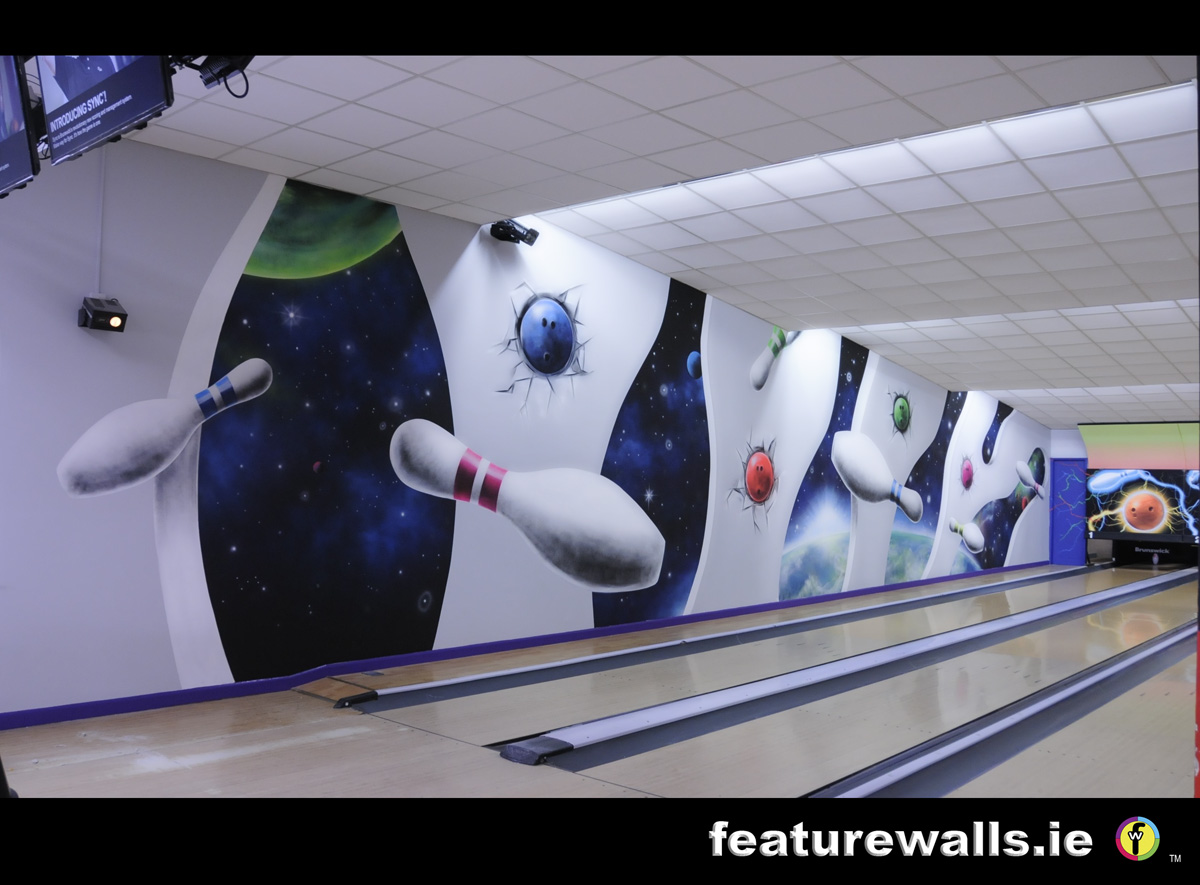The image showcases a display from the brand "FutureWalls.ie," identified by a distinctive "W" symbol in the bottom right corner set against a vivid yellow background, surrounded by a colorful logo featuring purple, red, green, and blue hues. The focal point of the image is an intricate and imaginative wall mural. This mural depicts bowling balls embedded in the white sections of the wall, simulating impacted areas with realistic damage. The artwork transitions from the terrestrial to the celestial, featuring elements such as Earth, outer space, and twinkling stars. Bowling pins are whimsically illustrated as if they are flying across the sky. At the base of the mural, bowling lanes can be seen, grounding the fantastical elements in a familiar setting. The upper section of the image captures the ceiling and the roof structure, while TV panels positioned at the top left display the ongoing bowling game, seamlessly integrating with the themed wall art.